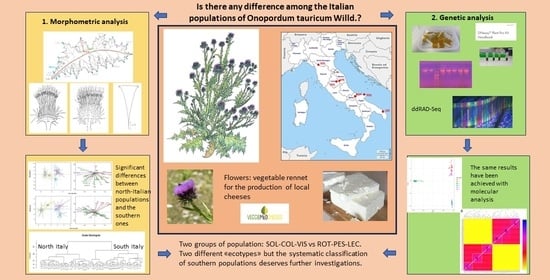The image is a detailed scientific diagram with a peach-colored background, likely from a study or teaching material concerning the geographical and genetic differences among Italian populations of the plant Onoportum tarucum wild. The centerpiece of the diagram features a map of Italy pinpointing the locations where this plant grows, surrounded by various images and text blocks. To the left of the map, there is a detailed drawing of the plant with multiple small purple flowers and a photograph of the same plant. Beneath these visuals, there is text noting, "flowers, vegetable rennet for the production of local cheeses," accompanied by an image of cheese bricks. The diagram also contains sections detailing "morphometric analysis," showing hand-drawn depictions of the plant's growth patterns and significant differences between northern and southern Italian populations. On the right side, under a green background labeled "genetic analysis," there are images potentially representing DNA sequencing data and scientific findings, stating that similar results have been achieved through molecular analysis. Additional referenced text mentions two groups of populations, differentiating between them with two ecotypes, and suggesting that the systematic classification of southern populations requires further investigation.